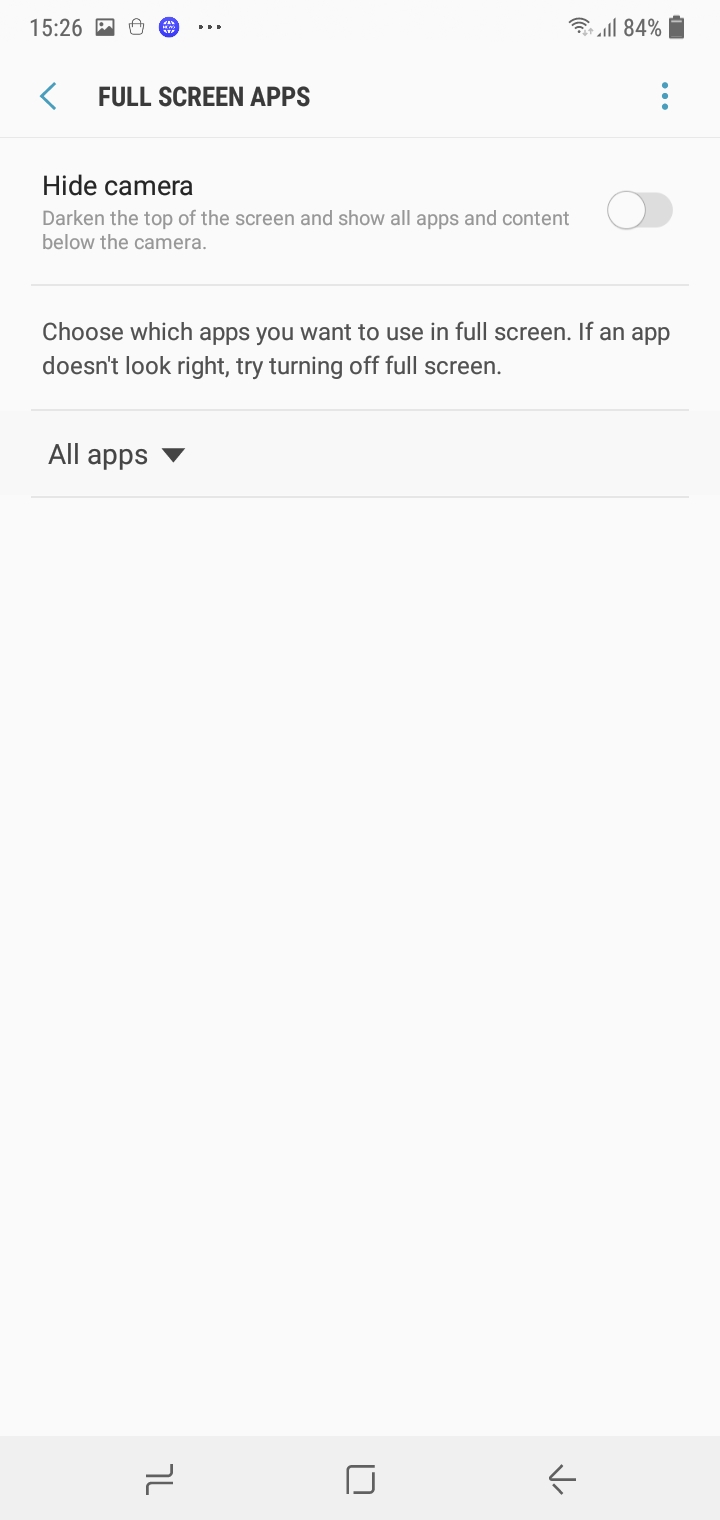The screenshot depicts the settings interface of a smartphone, specifically the "Full Screen Apps" section. The time displayed is 15:26, and various status icons indicate full Wi-Fi and cellular signal strength, along with an 84% battery level. The battery icon is prominently visible. 

At the top left, there's a back arrow icon, accompanied by the text "Full Screen Apps." Adjacent to this is a three-dot menu icon, suggesting additional options. The interface also includes instructions and options for managing full-screen settings: "Hide camera," "Darken the top of the screen and show all apps and content below the camera." A toggle switch for these settings is currently set to "off."

Further settings allow users to choose which apps to use in full-screen mode, with a note advising that if an app doesn't display correctly, users should try turning off the full-screen option. Below this, there is an expandable section labeled "All apps," indicated by a down arrow, which, when tapped, would reveal a complete list of applications available on the device.